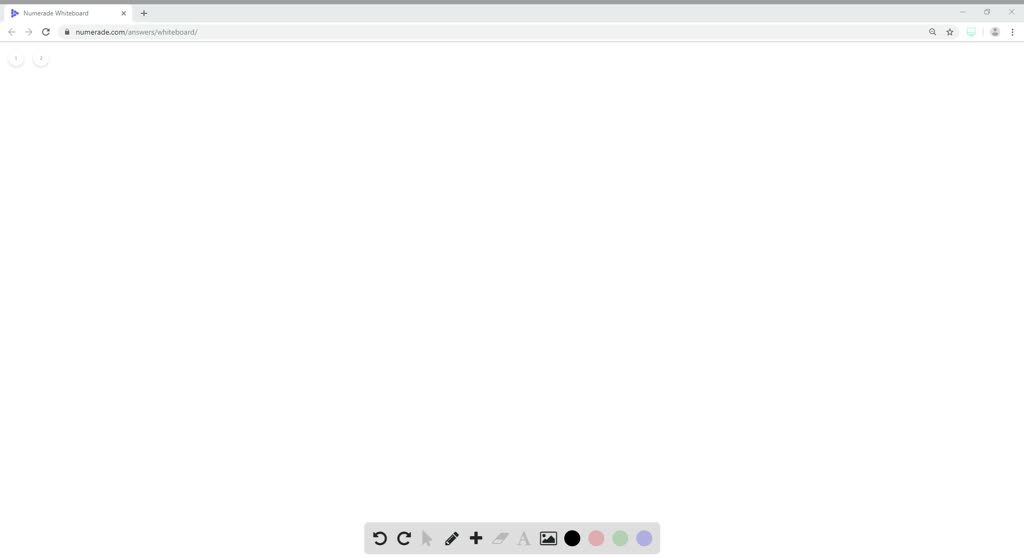A detailed depiction of a Chrome-like web browser window open on a whiteboard website named "Numenad" or a similar name. The browser interface, which appears to be a slightly unusual version of Chrome, features the familiar address bar, bookmarks star button, and a single open tab. The whiteboard workspace itself is entirely blank, with no drawings or writings currently visible. Along the bottom of the browser, a toolbar displays various tools such as a marker and eraser, allowing the user to select different functionalities to interact with the whiteboard. Additionally, options for changing the background color are visible, including the option to switch to a black background with white text. The window's title bar is typical of a Windows operating system, complete with the standard window management controls.